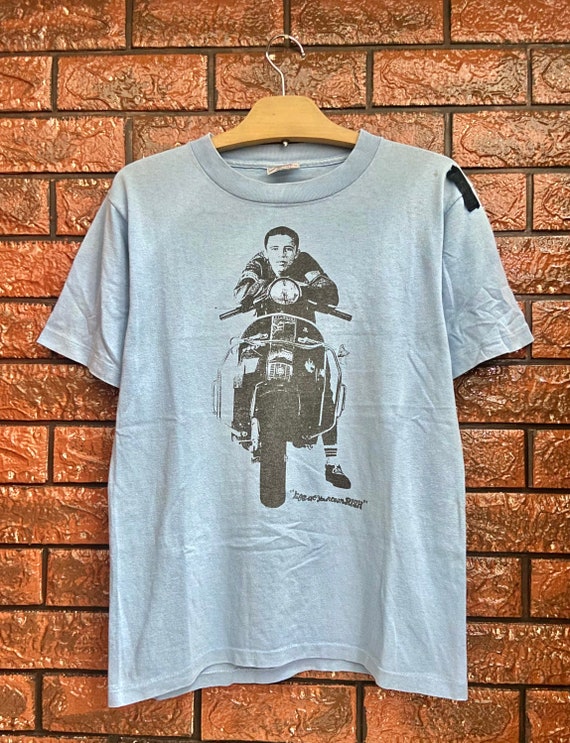In this image, we see a vintage-style t-shirt hanging against a nude, brown brick wallpaper background. The t-shirt, which is pale light sky blue, is displayed prominently centered in the photo, nearly occupying the entire frame in portrait mode. It hangs from a light brown, metal and wooden hanger attached to a protruding hook on the wall. The t-shirt features a black and white graphic of a young man on a motorbike, viewed head-on. The man, appearing to come from a 1950s era, has short dark hair and wears a black leather jacket. He is leaning his elbows on the handlebars of the motorcycle, and his intense gaze is directed straight at the viewer. Adjacent to the motorcycle graphic, there is text, though the specific words are not clearly visible. The overall image captures a striking, retro aesthetic.